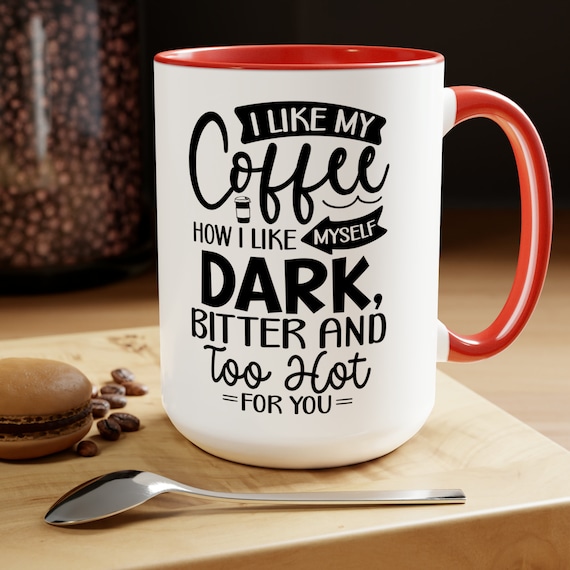This indoor photograph showcases an artfully arranged scene on a light brown wooden board, possibly set atop a matching tabletop. Central to the image is a distinctive coffee mug, predominantly white with a vibrant red handle, interior, and top lip. Adorned with whimsical text, the mug declares, "I like my coffee how I like myself: dark, bitter, and too hot for you," in a mix of black print and cursive. Positioned to the right of the mug, a silver spoon lies upside down. On the left side, a chocolate macaron and a scattering of brown coffee beans add a touch of indulgence. In the background, a glass jar filled with more brown beans is partially visible on the left, contrasting with the blacked-out right side, adding depth and interest to the composition.